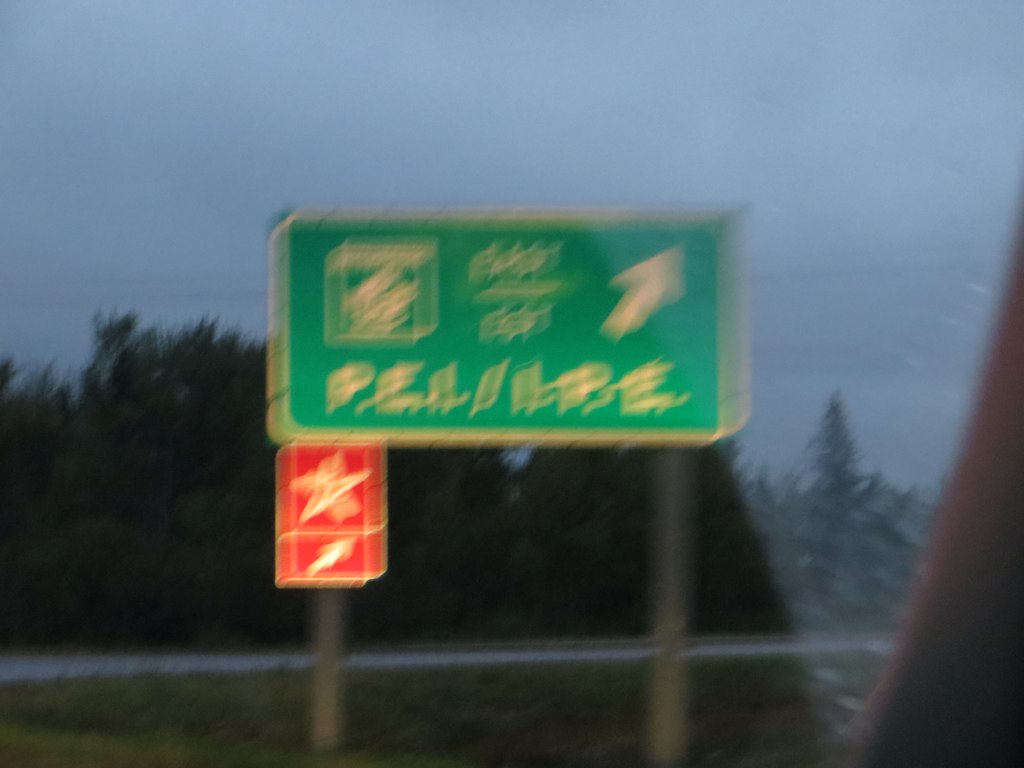The snapshot, taken through the window of a moving vehicle, captures a blurry outdoor scene bathed in gray-blue sky and flanked by a dense arrangement of tall trees, some possibly dusted with snow. Central to the image is a large, rectangular green road sign with white lettering, mounted on two metallic poles. While the text is mostly indistinct due to the blur, "P.E.I." and directions pointing northeast can be vaguely identified. Below the green sign, a smaller red sign with a white star and arrow is visible, which might indicate a logo or direction pointer, possibly relating to a gas station. Blurry curvatures suggest the presence of the vehicle window, and a white line across the bottom hints at a distant road.